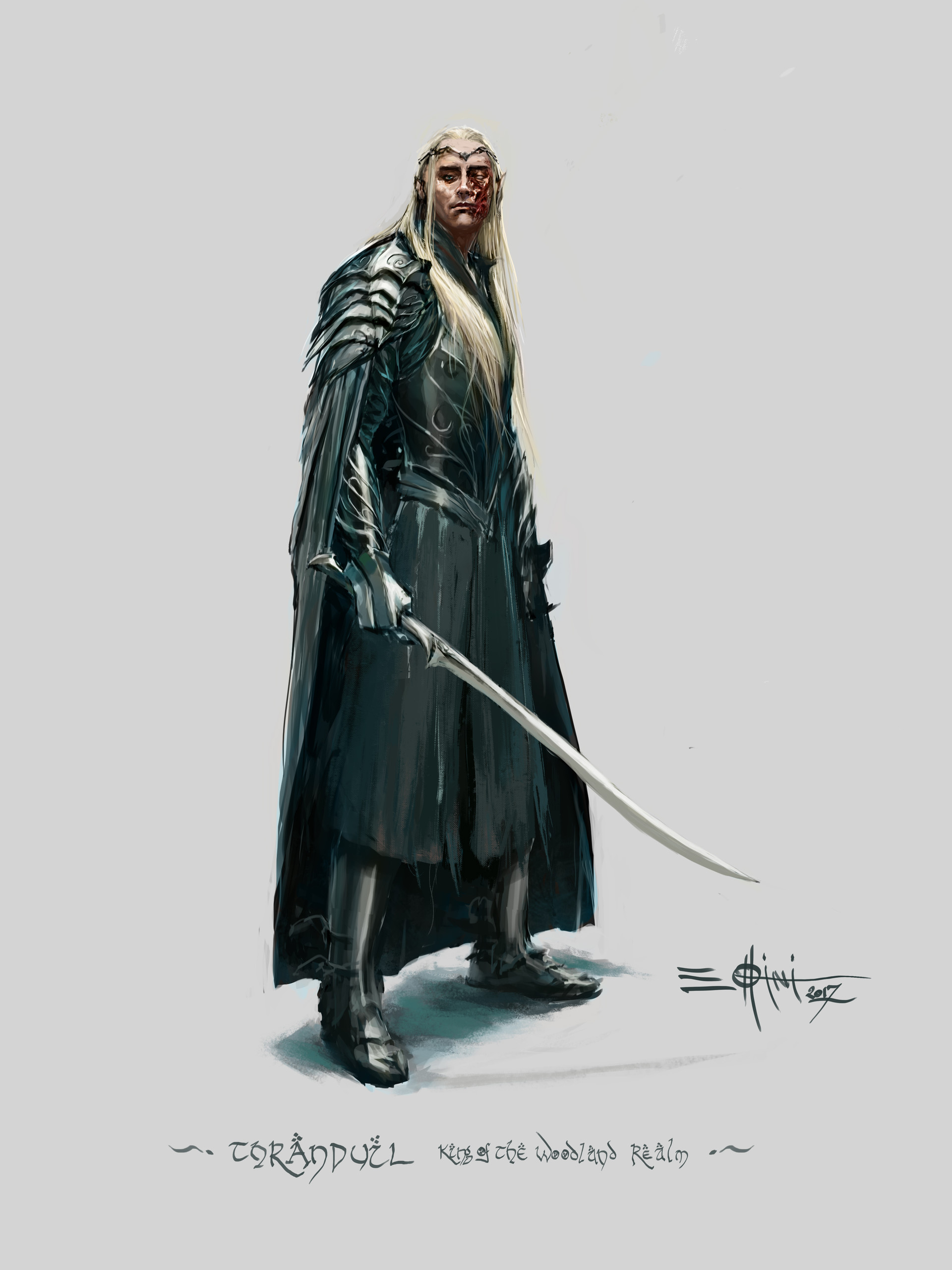This detailed illustration depicts a fantasy character who could easily be from J. R. R. Tolkien's "The Lord of the Rings" universe, reminiscent of an elfin warrior. The character, named Thranduil, King of the Woodland Realm, is rendered in a pen and ink style or computer-generated artwork. He commands attention with his long blonde hair and a black leather cape that extends to the ground. The cape also features layers of shoulder epaulets. He stands with a majestic, slightly wounded or scarred face, looking directly at the viewer. His attire includes a leather jacket-like tunic that resembles a medieval dress, complemented by black boots. He wields a lethal, swooping sword in his right hand, while his left hand is obscured. His head is adorned with a vine or headband-like crown. There are black, stylized letters at his feet that read "Thranduil, King of the Woodland Realm," along with an artist's signature nearby. The overall image evokes a somber, yet regal, warrior presence.